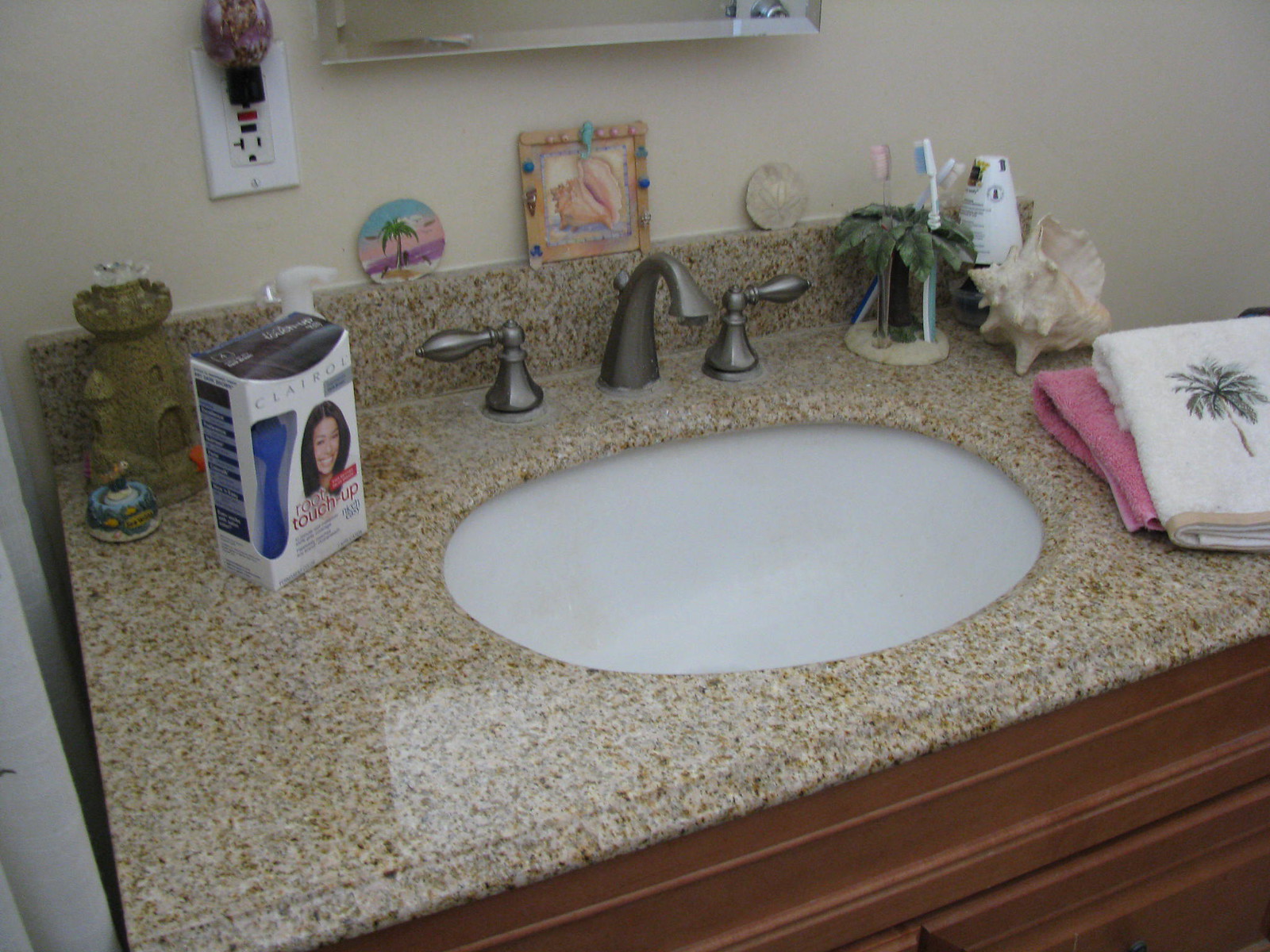This image captures a detailed close-up of a bathroom sink area. The sink is installed atop a dark brown framed countertop, featuring hints of two cabinet doors beneath it. The countertop is crafted from granite, presenting an intricate pattern composed of brown, yellowish-gold, gray, and white specks. To the right, two towels are neatly stacked, with the bottom one in pink and the top in white, adorned with a green palm tree logo. Adjacent to the towels stands a decorative palm tree figure and several toothbrushes. Nearby, a white, cone-shaped air freshener and a large shell rest on the countertop. The dark gray faucet and handles are centrally positioned. Above the sink, there are a few circular images and a small, square-shaped framed picture. To the left side of the countertop, there is a white box labeled "Touch Up," featuring an illustration of a woman with black hair on the front. This box has a dark gray top. Additionally, a white electrical outlet is mounted on the wall, which is painted in a muted gray color, completing the scene.